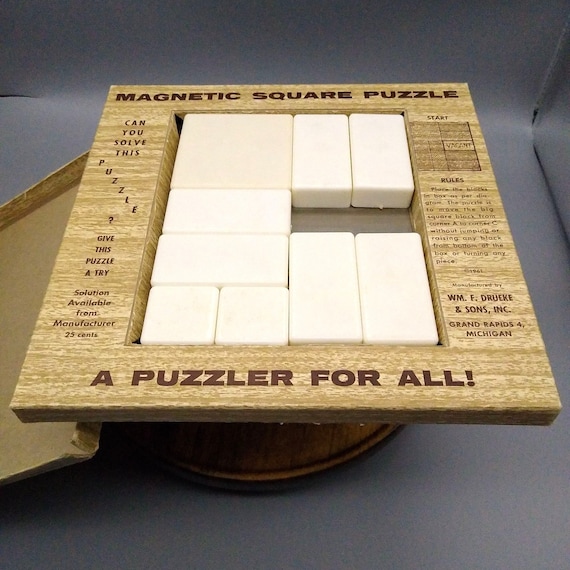The image features a wooden frame containing white tiles of varying sizes. At the top of the frame, in bold letters, is the title "Magnetic Square Puzzle." Below, the phrase "A Puzzler for All" is prominently displayed. On the left side of the frame, a block of text reads, "Can you solve this puzzle? Give this puzzle a try. Solution available from manufacturer. 29 cents."

Within the frame, tiles are arranged in a grid. A square tile is positioned on the left, while longer, skinnier tiles are placed along the right side and bottom. Notably, there is a single space left vacant within this arrangement. The entire setup rests on a gray surface.

Additional instructions and rules are written along the right side of the frame, explaining how to start the puzzle and emphasizing where the vacant space should be located.